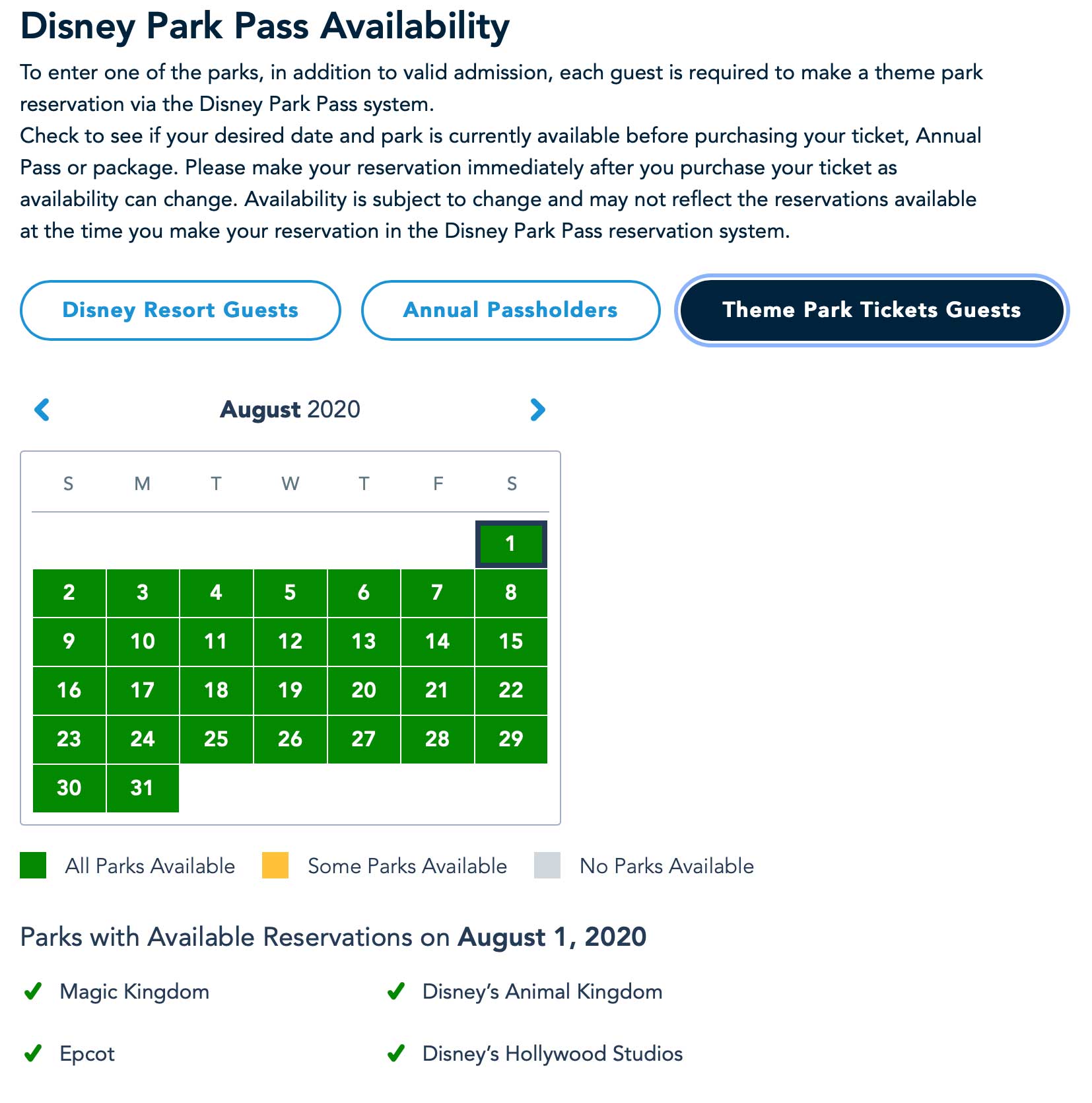The image displays a webpage with a white background and predominantly black text, indicating its critical information. At the top half of the page, in bold black text, it reads "Disney Park Pass Availability." Below this header, a detailed instruction informs guests that to enter any Disney park, a valid admission and a theme park reservation via the Disney Park Pass system are required. The text further advises guests to check the availability of their desired date and park before purchasing tickets. It also emphasizes that Annual Pass or Package holders should make their reservations immediately after purchasing tickets, as availability can shift rapidly.

The lower half of the page features a calendar for August 2020. All displayed dates are marked with green boxes, signalling open reservation slots. Above the calendar, the month "August 2020" is stated in bold text. Beneath the calendar, another piece of information reads "Parks with Available Reservations on August 1st, 2020," followed by a list of the parks: Magic Kingdom, Epcot, Disney's Animal Kingdom, and Disney's Hollywood Studios.